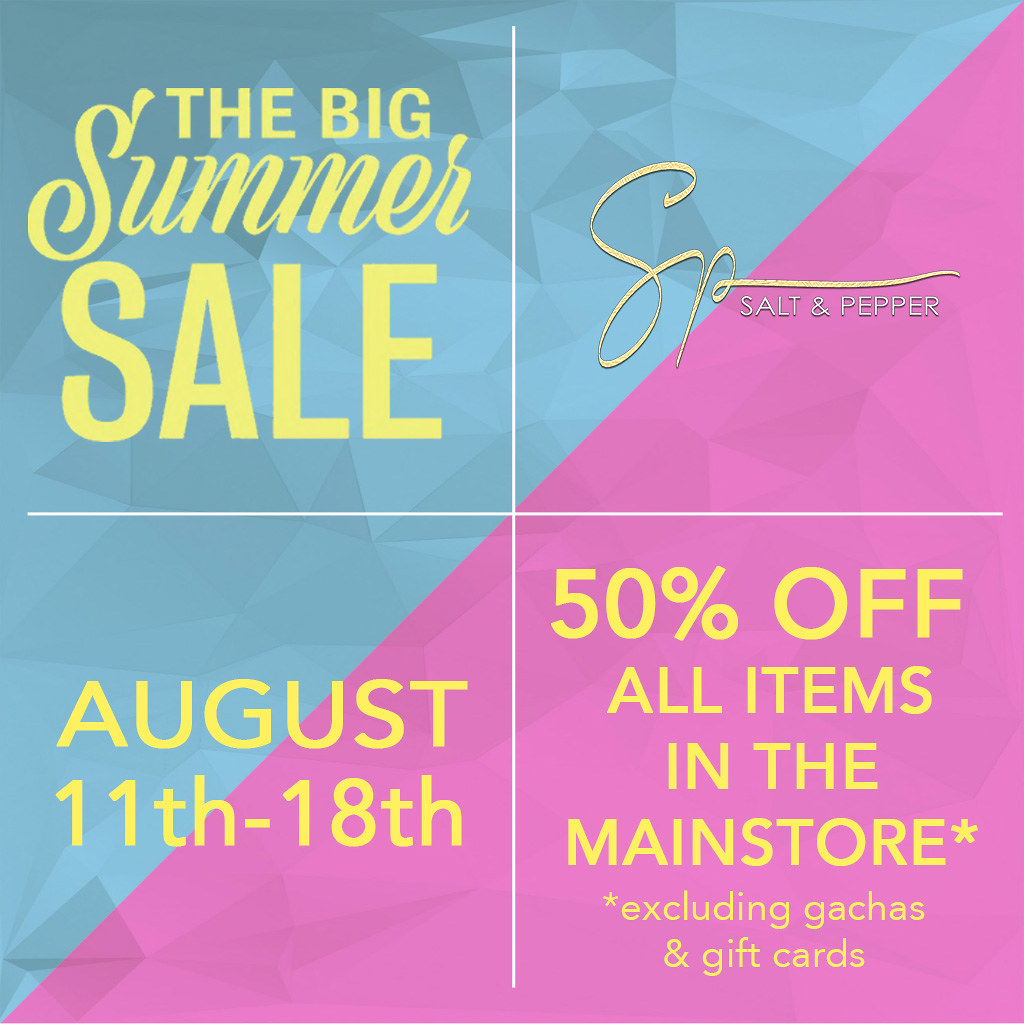This vibrant square advertisement is divided into four white-bordered quadrants with a diagonal line separating a bluish left triangle from a pinkish-purple right triangle. Each quadrant contains yellow text that highlights key details: the upper left quadrant announces "The Big Summer Sale" in bold yellow print, while the upper right quadrant features the scripted "SP Salt and Pepper." The lower left quadrant lists the sale dates as "August 11th to 18th." In the lower right quadrant, it proclaims "50% off all items in the main store," with an asterisk noting that the discount excludes gotchas and gift cards.